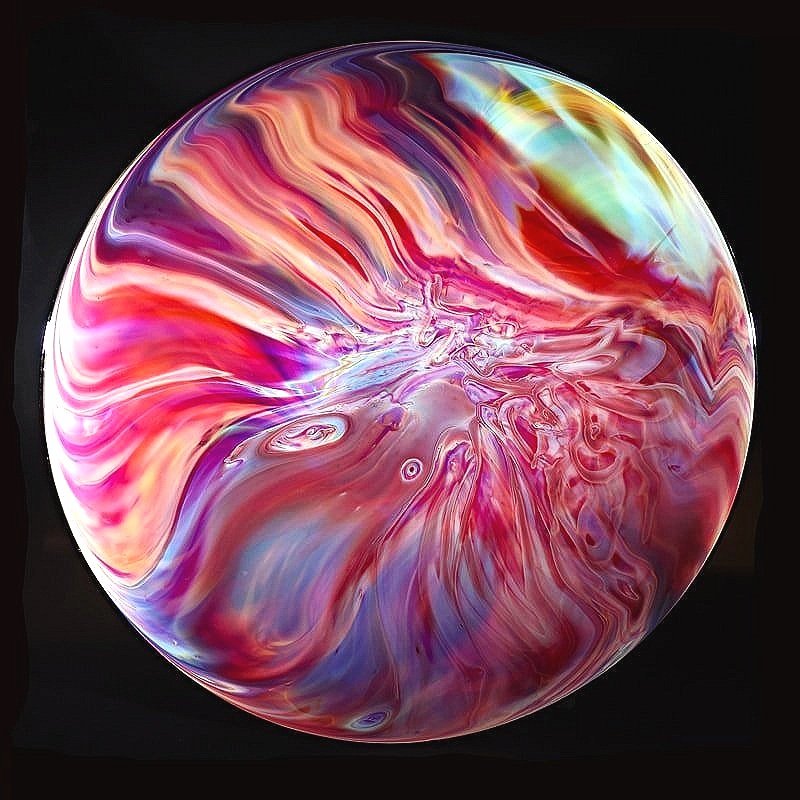The image features a striking circular object set against a black square background. This central orb exudes a mesmerizing appearance, reminiscent of a marble or a flat view of a bowling ball. It showcases a vibrant mix of colors, predominantly red, pink, and white, with additional shades of purple, blue, maroon, yellow, and orange. These colors swirl together intricately, creating a dynamic, marble-like effect. Notably, the swirl patterns are chaotic and intermingled in the middle, while the outer regions, especially the upper left and middle left, display more parallel and organized lines. Light seems to project onto the orb from the left side and the upper right portion, giving it a subtle, sunlit look, enhancing the overall depth and dimension. The artistic effect is that of red paint swirled through a white base, creating an illusion of colorful material oozing out from the center.